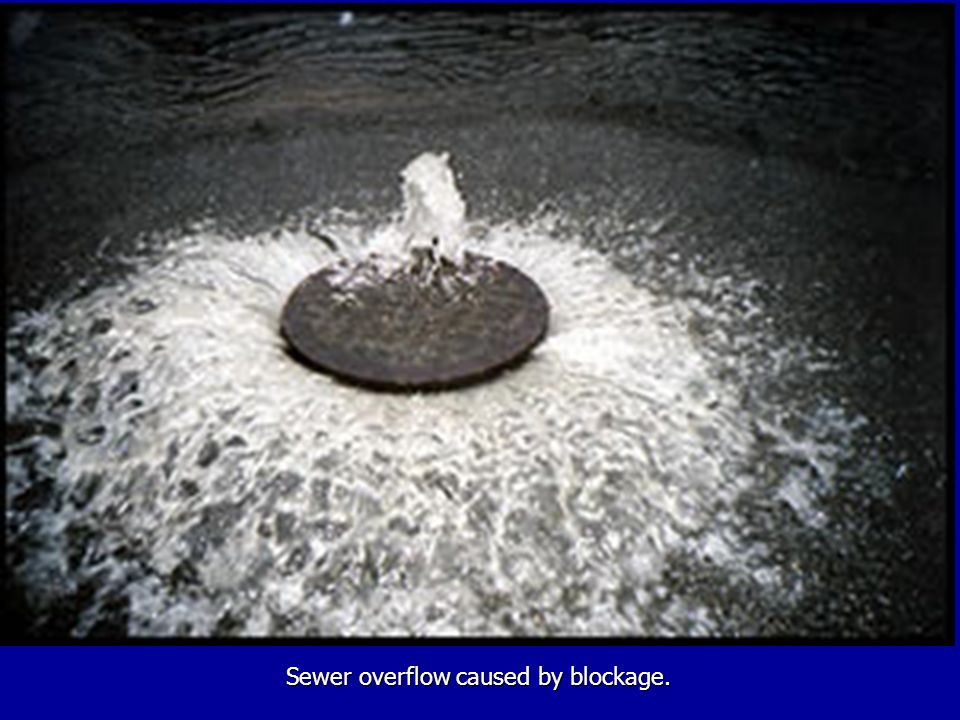The image depicts a low-resolution, black-and-white photograph capturing a sewer overflow caused by a blockage. At the center of the photograph, a manhole can be seen with water gushing out radially, resembling a short, wide fountain approximately three feet high. This water appears white against the grayscale backdrop of the surrounding road. The road surface around the manhole is dark, transitioning to a textured, built-up area towards the top of the image, which is similarly dark and striated. There are no people present in the scene. Beneath the image, a bright blue bar with white text declares, "Sewer overflow caused by blockage." The overall appearance and the style of the text suggest that the image may be sourced from an educational website or slideshow intended to illustrate sewer-related issues.